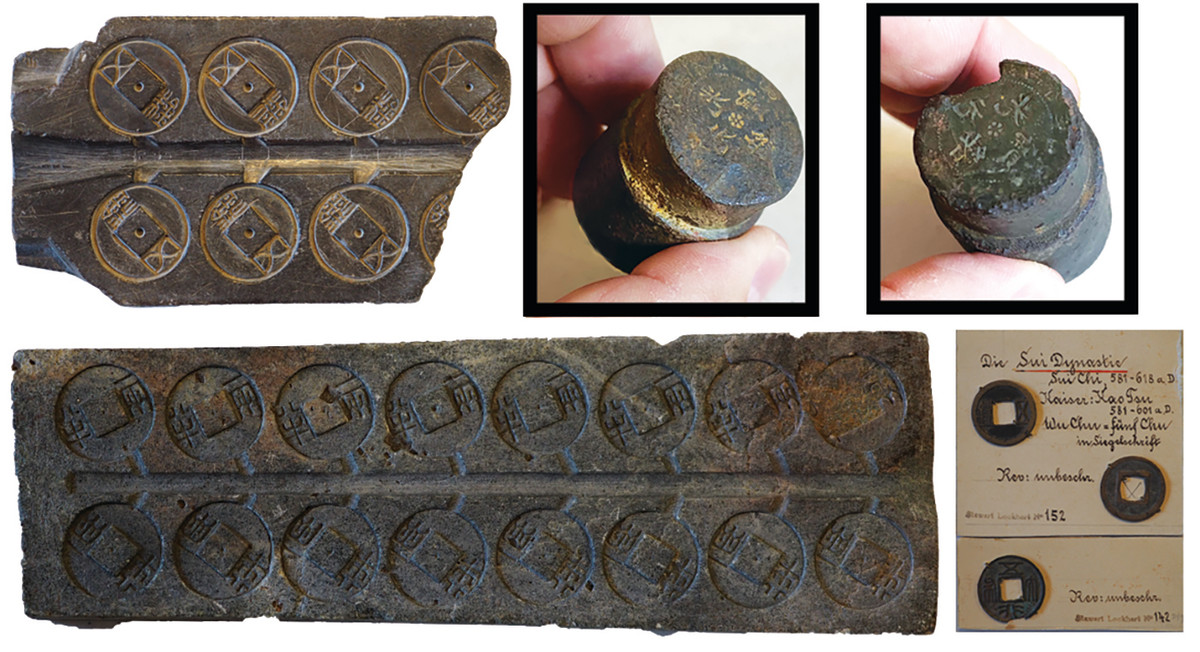The collection of images showcases the intricate process of traditional Japanese coin making. At the top, we see a series of three photographs. The first image features a mold, possibly made of rock or iron, that allows for the mass production of circular coins with distinctive square holes in their centers. To the right of this mold are two close-up images of hands holding metal stamps used to impress designs or characters onto the coins. Below this row, the first image shows a long, metallic bar with two rows of coin-shaped outlines, presumably part of the minting process. To the right, the final image displays a set of fully produced coins, round with square holes in the middle, bearing what appears to be Japanese or Chinese characters. These detailed photos collectively depict the craftsmanship and tools involved in the coin-making process.